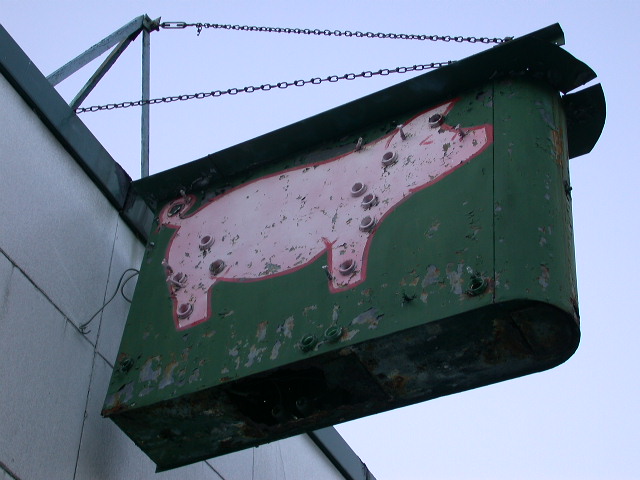This photograph features a worn-down restaurant or business sign depicting a bright pink pig outlined in an even brighter pink, positioned on a green, metallic, rectangular sign with rounded edges on the right side. The paint is visibly chipped, revealing rusted metal underneath, and there are numerous circular holes across the sign, possibly remnants of old neon tubes. The sign hangs by two chains from a triangular metal piece extending perpendicularly from the roof's façade, which consists of a gray cinder block wall with a black cornice along the top edge. The sky behind the sign is a clear blue, and wires can be seen protruding from the back of the sign, contributing to its dilapidated and poorly maintained appearance.